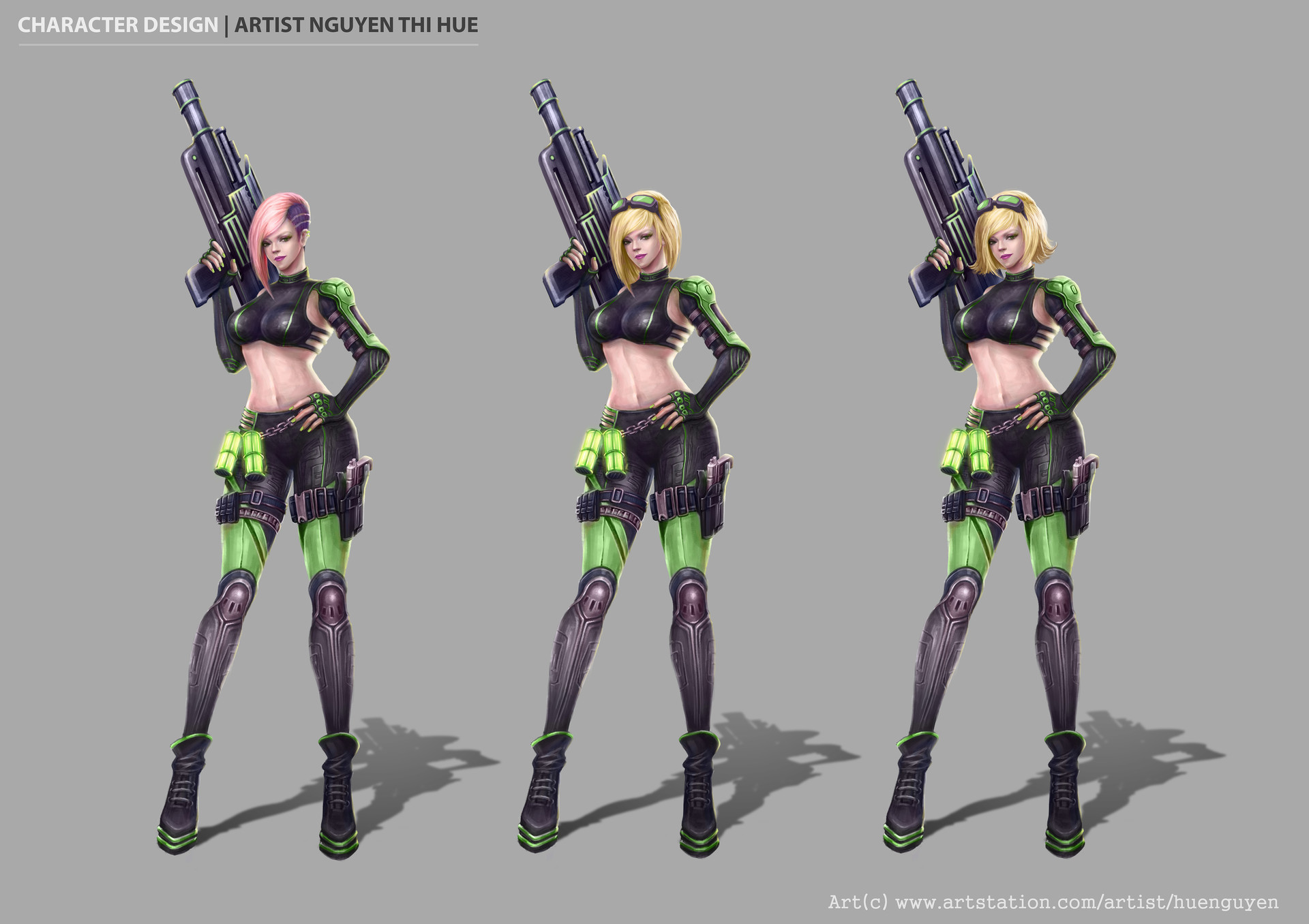The image titled "Character Design" by artist Nguyen Thi Hue showcases three intricately designed female characters, each presenting unique yet subtly distinct features. At the top left of the image, "Character Design" is written in white text, with “artist Nguyen Thi Hue” inscribed in black below. These characters are futuristic and sci-fi themed, sharing the same black and purple armored suit accessorized with a large, blue-and-green outlined gun, which they carry over their right shoulders. 

The character on the left is distinguished by her pink hair, styled with a fade on the left side featuring two lines. She also sports purple boots and additional fighting accessories strapped to her right thigh. The middle character exhibits golden blonde hair adorned with green goggles and carries the same futuristic weapon. Lastly, the character on the right, similar to the middle one, has short blonde hair with a bob cut and green goggles perched atop her head. 

At the bottom right corner of the image, there is a copyright notice followed by "www.artstation.com/artist/HueNguyen" written in white text. The collective apparel includes a form-fitting black top with a mesh back, tight black pants with green accents on the mid-thigh, and black platform shoes with green bands, highlighting their sleek and advanced design.